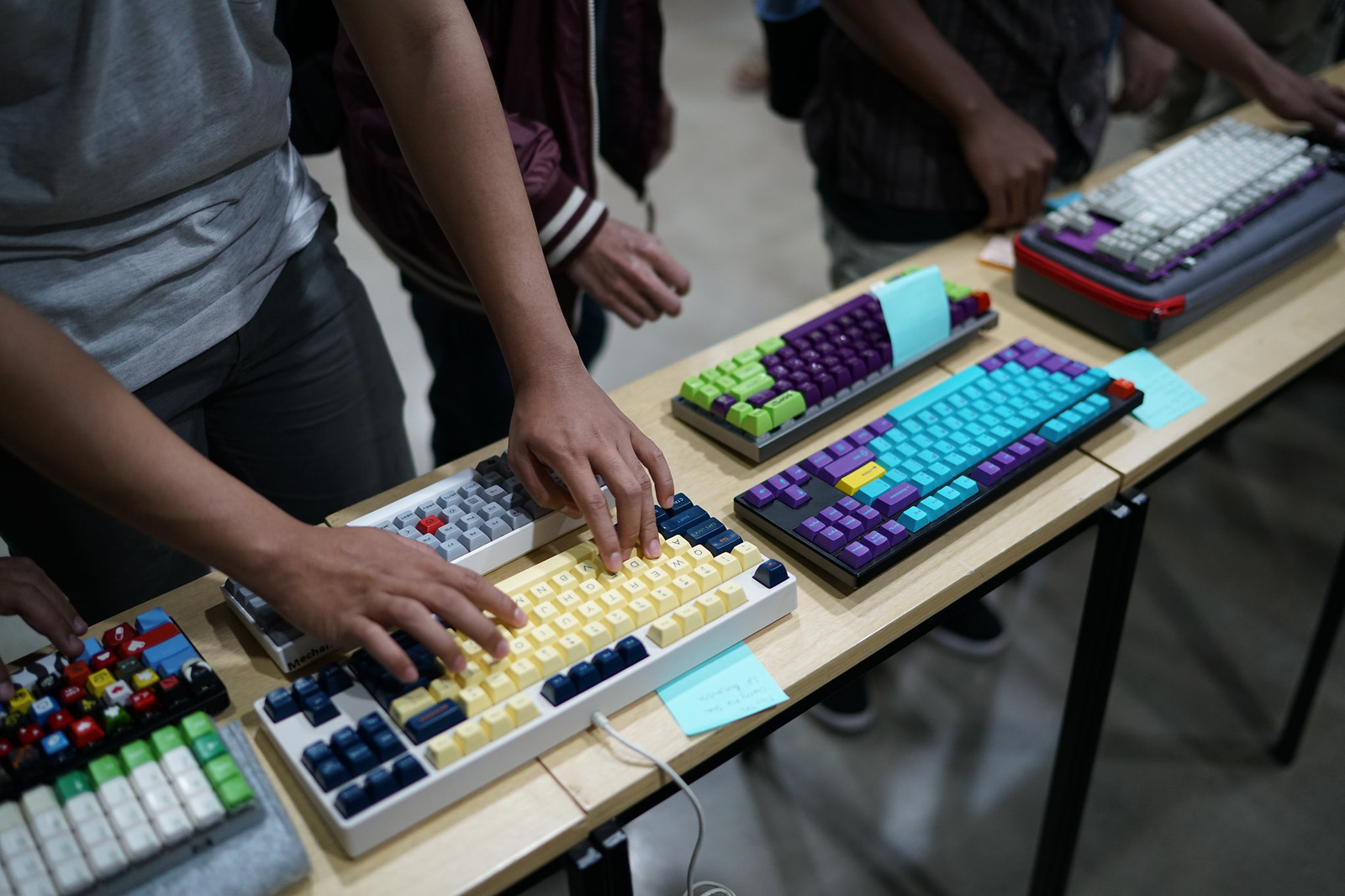In this indoor photo, a long, narrow table composed of connected, rectangular segments with black metal legs and a light wooden top supports a diverse array of seven colorful computer keyboards. Each keyboard has a small blue post-it note beside it. The keyboards vary widely in color combinations, including black with purple and teal keys, white with blue keys, and multicolored arrangements. A person with a medium dark complexion and short fingernails, dressed in a gray shirt and dark pants, is typing on a vibrant black, white, and cream keyboard. To his right, two individuals with slender arms and similar medium dark complexions also engage with the keyboards. While their faces are not visible, their body language shows active interest. The gray flooring of the room, along with the eclectic spectrum of keyboards, adds to the detailed scene of people attentively interacting with technology.